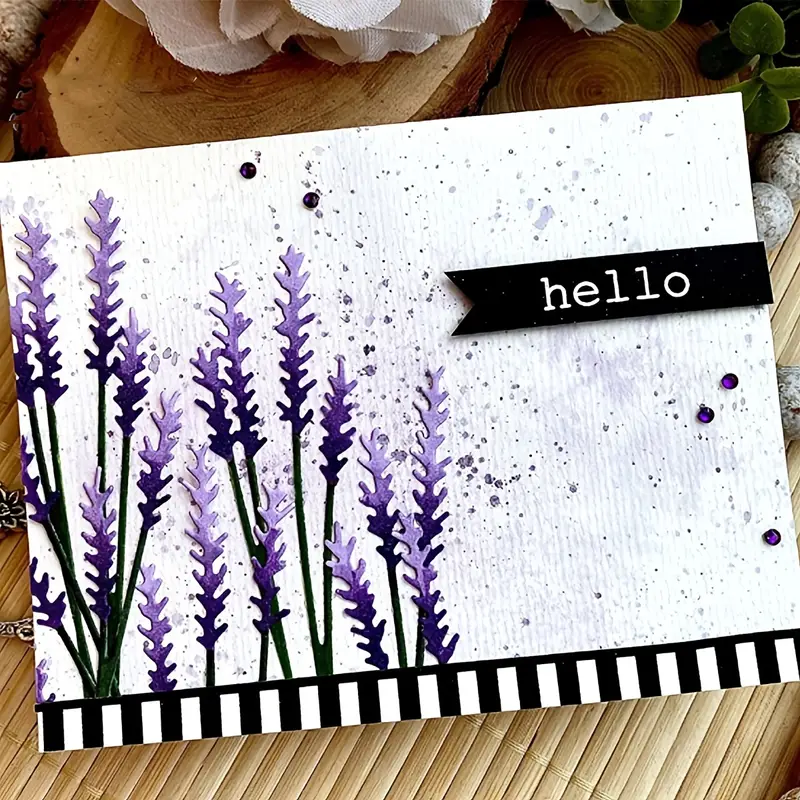The image showcases a white note card placed centrally on a brown bamboo mat. The card is held up at the top by what appear to be brown wooden discs. The card features an intricate design with long-stemmed flowers in shades of light and dark purple spanning the left side. The right side of the card has a black ribbon with the word "hello" written in white on it. The card is also adorned with speckles of purple and gray, providing a delicate, scattered pattern. At the bottom of the card, there's a black and white checkered strip, reminiscent of piano keys. The colors in the image predominantly include light tans, darker browns, lavender, white, and black, creating a harmonious and aesthetically pleasing look.